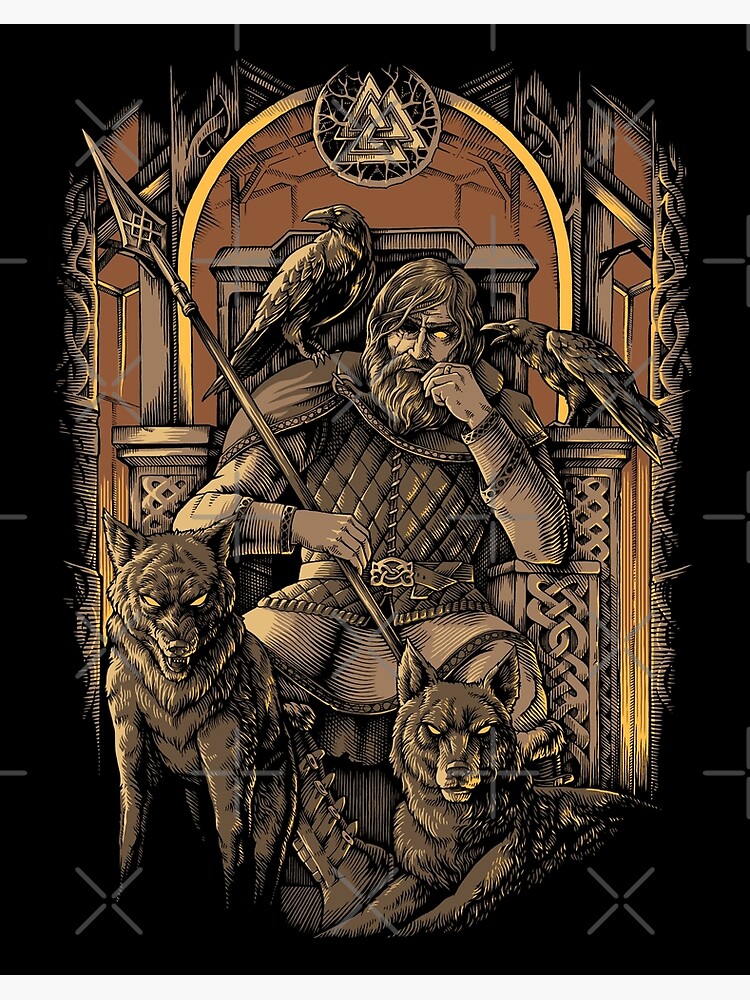In the image, we see a detailed drawing of a warrior or knight from ancient times, seated on an elaborately designed throne. The man has long, straggly hair, a beard, and a long mustache. He has one black eye on the left side of the image and a yellow or white eye on the right, lending him a mysterious or otherworldly appearance. He is clad in shades of muted grays and browns, with a touch of yellow in the throne's arch behind him and around some details. 

The warrior is leaning on the throne's armrest with his left hand near his face, while his right hand holds a long spear or sword that stretches across his body. Two imposing ravens accompany him; one perches on his left shoulder, and the other rests on a part of the throne near his head to the right.

At the feet of the throne are two black wolves with piercing yellow eyes, enhancing the menacing aura of the scene. The wolf on the left is lying down, appearing calm yet alert, while the other on the right is sitting on its haunches, teeth bared in a snarl. The background of the drawing is predominantly black, providing a stark contrast that accentuates the muted colors and intricate details of the central figures and their surroundings. Above the warrior’s head, there is an interwoven circle consisting of three triangles, adding to the mystical or symbolic elements of the piece.